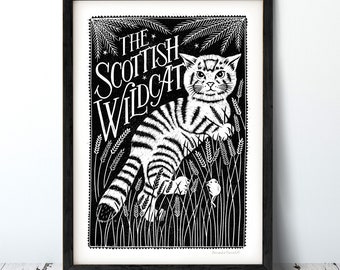This detailed descriptive caption combines and refines the provided captions:

The image features a framed artwork with a black frame and a white mat, set against a white background likely on a wooden surface. The central image has a black background, showcasing an intricate drawing or print of a Scottish Wildcat in black and white. The wildcat, adorned with black stripes, stares directly at the viewer, exuding a poised presence. Surrounding the wildcat are delicate, white sprigs resembling wheat or barley, growing upwards in graceful, curved lines from the bottom and corners of the frame. Noteworthy is a small mouse climbing one of these stalks in the bottom right corner, unnoticed by the watchful wildcat. The title, "The Scottish Wildcat," is written in a curvy, handwritten font at a 45-degree angle from the middle left to the upper middle portion of the image, adding an elegant touch to the composition.